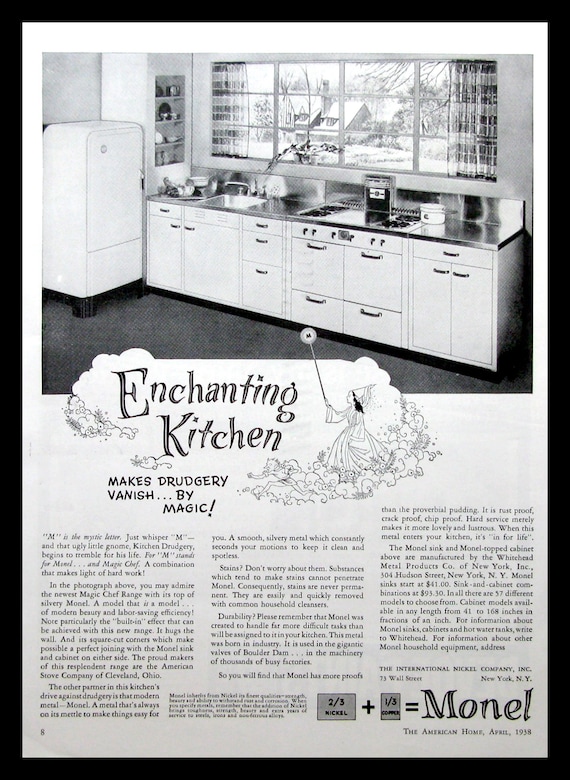The advertisement flyer showcases a vintage, black and white kitchen from the 1950s or 1960s. The focal point is the captivating tagline, "Enchanting kitchen makes drudgery vanish by magic," displayed prominently along with an image of a fairy or lady holding a sign featuring the letter 'M'. The flyer promotes the latest model of the Magic Chef range, emphasizing its silvery top and modern beauty combined with labor-saving efficiency. The range, produced by the American Stove Company of Cleveland, Ohio, is highlighted for its built-in effect and perfect alignment with the mantel sink and cabinets. The scene presents a comprehensive view of the kitchen, detailing appliances such as the refrigerator in the upper left, the counter with the sink, and a stove on the right—all framed by a large, 12-pane window that offers a glimpse of a possibly snowy landscape outside. This advertisment, featured in the April 1938 edition of "The American Home" magazine, underscores the enchantment of a modern kitchen that simplifies household chores.